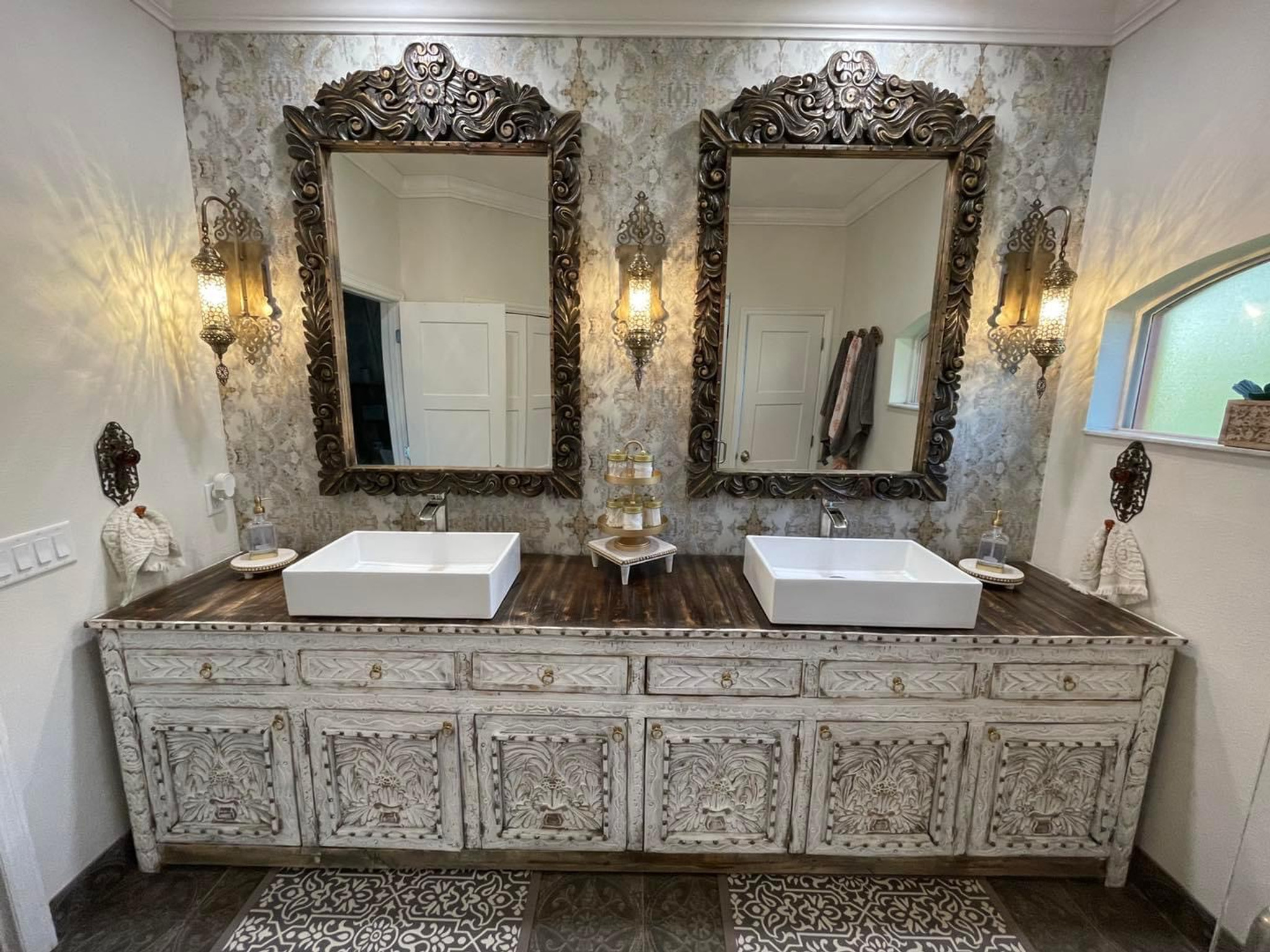This photograph depicts a luxurious, high-scale indoor bathroom. Dominating the image is a long, ornate wooden countertop with a rustic white-painted front. Below the countertop, there are six cabinet doors and an array of slender rectangular drawers, each fitted with a central knob. The countertop houses two modern square-shaped sinks, one on each end, with matching soap dispensers in little white bowls on either side.

Above the sinks are two large rectangular mirrors, each encased in an intricately designed, heavy-looking metal frame with swirls and ornate lines. Between and beside each mirror, a series of three illuminated, ornate lights hang from the wall, casting a warm glow on the scene. Adding to the elegance of the setting, a collection of smaller bottles is neatly arranged in a holder placed centrally between the two sinks. The walls are adorned with a wallpaper that harmonizes with the cabinet's rustic aesthetic, completing the sophisticated ambiance of the bathroom.